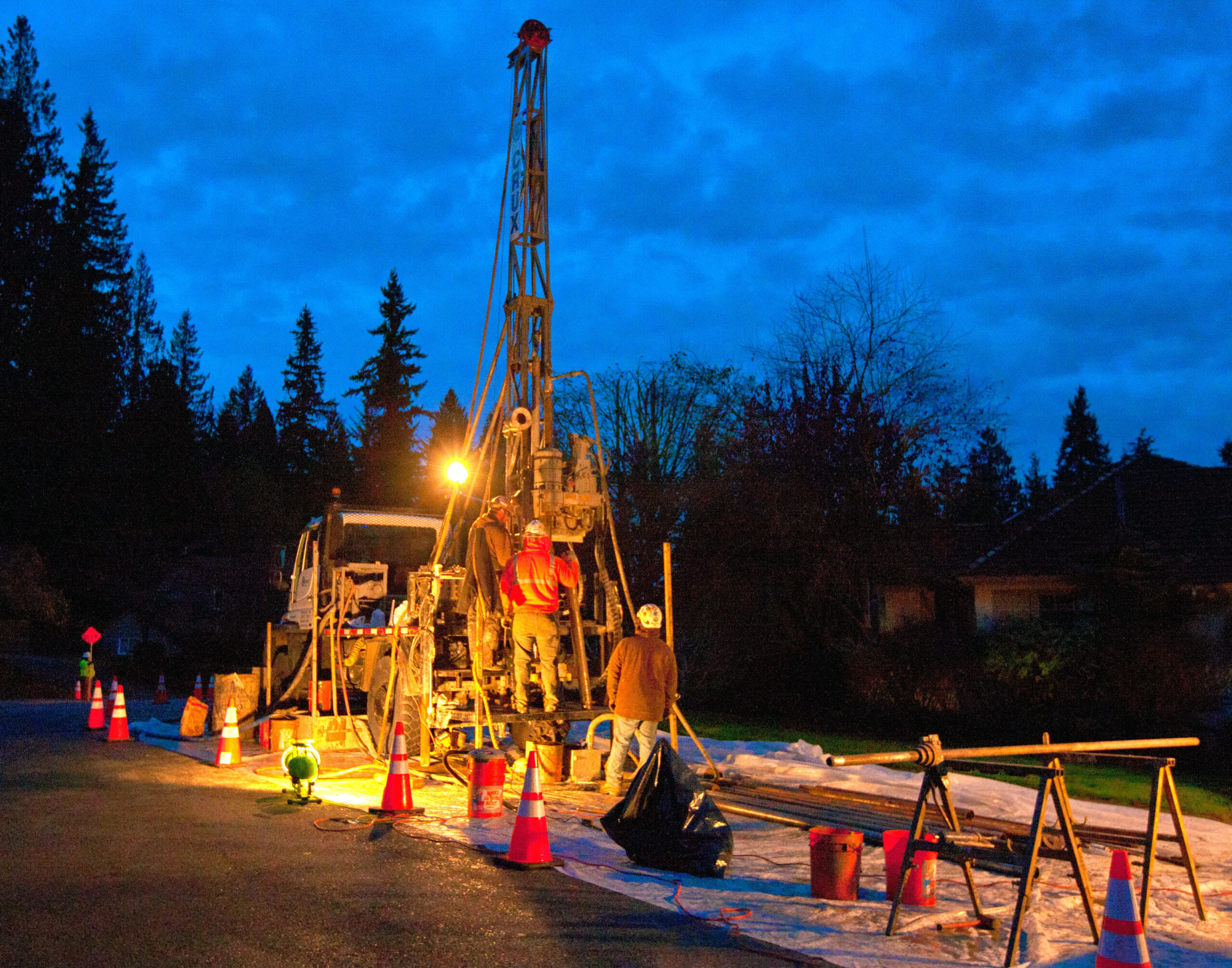In this nighttime photograph, captured under a cloudy sky with rows of trees and a cozy house on the right, we see a busy construction scene focused on a large drilling machine mounted on the back of a semi-truck labeled "Crux." The machine, which resembles a mini tower with a red horn atop and hoses trailing from it, dominates the center of the image, extending to the top edge. Flanking the drilling machine are two workers on the platform, dressed in brown and orange jackets, and wearing white helmets. Another worker, also in a brown coat and white helmet, stands at the base, while a fourth man in a bright yellow jacket and hard hat holds an orange caution sign to the left.

The area is enclosed by orange traffic cones and a white tarp spread across the road, indicating a secure work zone. Scattered around the workers are wooden planks and metal planks, adding to the construction elements. Illuminating their workspace, a spotlight shines from the right side, and the truck itself emits a glow, making the scene clearly visible despite the late hour.